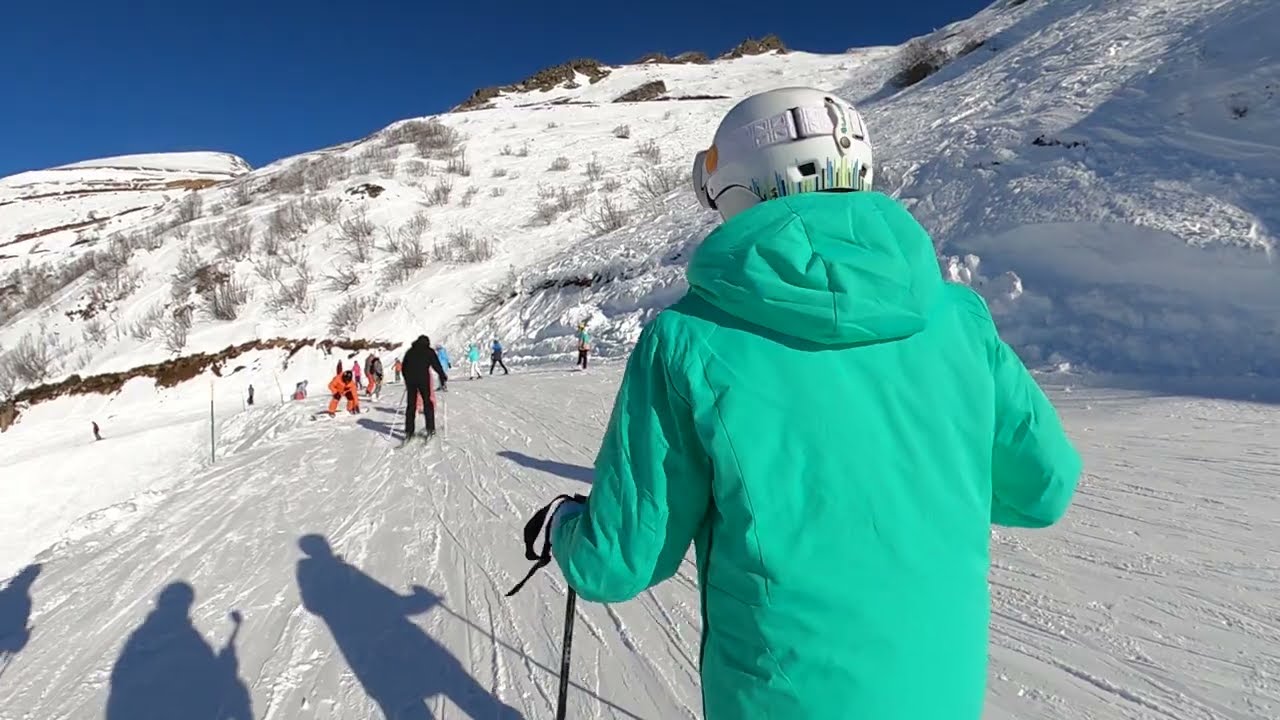This outdoor photograph depicts a bustling ski area on a clear, sunny day with numerous people skiing on a snow-covered slope. Centered in the foreground is the back of a skier dressed in an aqua or turquoise jacket with a hood and wearing a white helmet. While the skier's face and exact actions are not visible, they are clearly holding a ski pole and potentially a selfie stick. Their shadow, along with two others, falls on the lower left corner, indicating the sun is shining from the upper right. The slope appears gentle, suggesting a beginner trail populated by several skiers, including children. Surrounding the skiing activity, the terrain transitions into snow-covered hills with rocky tops and dead trees. The deep blue sky overhead contrasts with the rugged, partly barren mountains, adding to the scenic beauty of this wintry landscape.